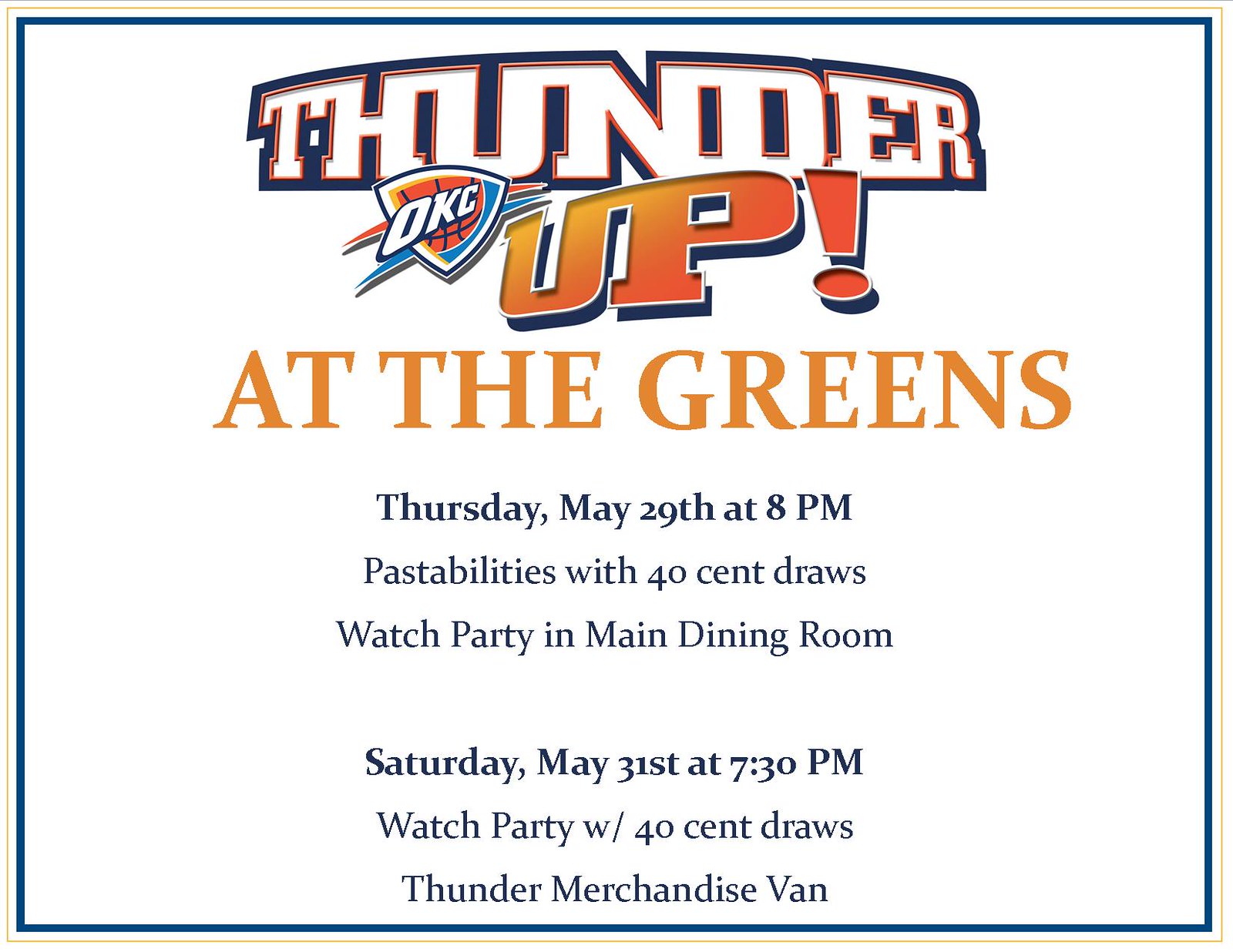The image is a poster advertising an event for the Oklahoma City Thunder. At the top, it reads "Thunder Up" in a stylish manner with the "OKC" shield logo featuring a basketball design beneath it. Followed by "At The Greens" written in all caps. The event details are listed below: "Thursday, May 29th at 8 PM: Pastabilities with 40 Cent Draws. Watch Party in Main Dining Room," and "Saturday, May 31st at 7:30 PM: Watch Party with 40 Cent Draws. Thunder Merchandise Van." The poster's background is white, encircled by a dark blue border and a thin light brown (or yellow-orange) outer border. The poster is slightly wider than it is tall. Textual details including date and times are in blue text, with the word "Thunder" in white text bordered by blue, and "Up" in orange text.